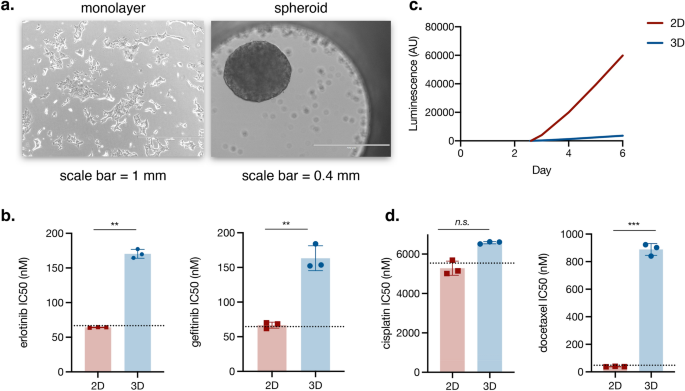The scientific infographic comprises a detailed array of figures showcasing various data visualizations. In Figure A, there are microscopic images labeled "monolayer" with a scale bar representing 1 mm, and "spheroid" with a scale bar of 0.4 mm. Figure B and Figure D are bar graphs featuring red and blue bars, illustrating comparative data, with the blue bars typically higher than the red. Figure C presents a detailed line graph where red lines represent 2D data and blue lines represent 3D data; the x-axis marks the days (0, 2, 4, 6) while the y-axis shows luminescence levels ranging from 0 to 8,000, with the 2D data peaking around 6,500 and the 3D data remaining near baseline levels. Throughout the infographic, visual elements such as shades of gray, blue, red, and black text are utilized to enhance clarity and emphasize critical data points.